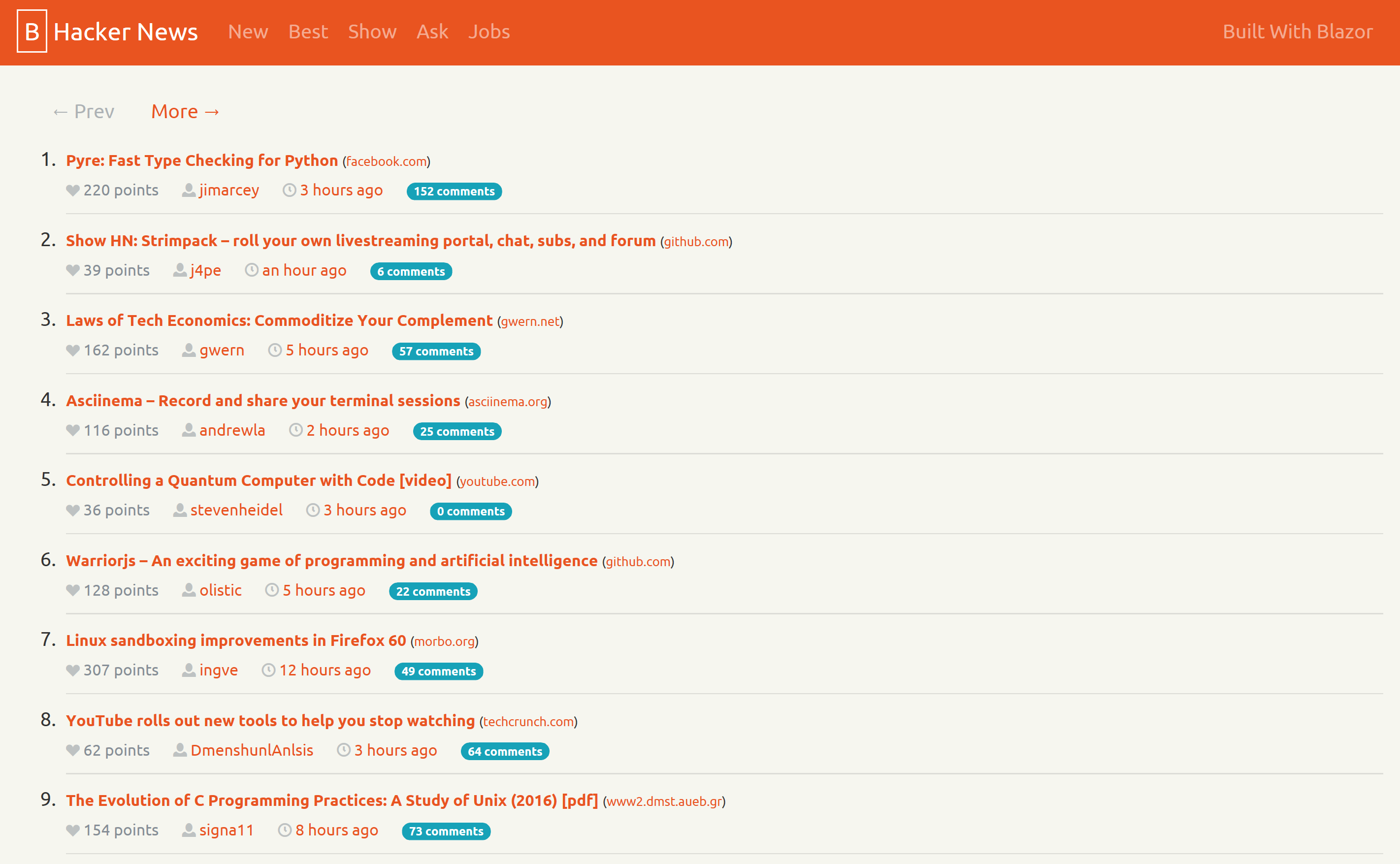The image is a screenshot from the Hacker News website. At the top, there is an orange navigation bar with the Hacker News logo in white. Accompanying options include "new," "best," "show," "ask," "jobs," and "built with Blazor." The bar also displays navigation links for "previous" and "more." Positioned next to the Hacker News logo is a bold 'B' inside a vertical rectangle with a white border.

Beneath the navigation bar, there are nine entries listed, each with an identifier ranging from 'up to 139,' followed by a description in orange text. The entries are:

1. "Pyre: Fast Type Checking for Python" - hosted on facebook.com, this entry has earned 220 points, was posted by J Marcy three hours ago, and has 152 comments.
2. "Show HN: Stream Pack - Roll Your Own Live Streaming Portal, Chat, Subs, and Forum" - found on github.com, it has received 39 points, was submitted by J for PE an hour ago, and has four comments.
3. "Laws of Tech Economics: Commoditize Your Complement" - available on govern.net, this entry has accrued 162 points, was posted by She Weren't five hours ago, and has 57 comments.
4. "ASCII NEMA: Record and Share Your Terminal Sessions" - on asciinema.org, the entry received 116 points, was submitted by Andrew LA two hours ago, and has 25 comments.
5. "Controlling a Quantum Computer with Code (Video)" - from youtube.com, this post received 36 points, was posted by Stephen Heidel three hours ago, and has zero comments.
6. "Warrior JS: Exciting Game of Programming and Artificial Intelligence" - available on github.com, it earned 128 points, was submitted by Ola Stick five hours ago, and has 22 comments.
7. "7 Linux Sandboxing Improvements in Firefox" - no further details are provided past this point in the list.